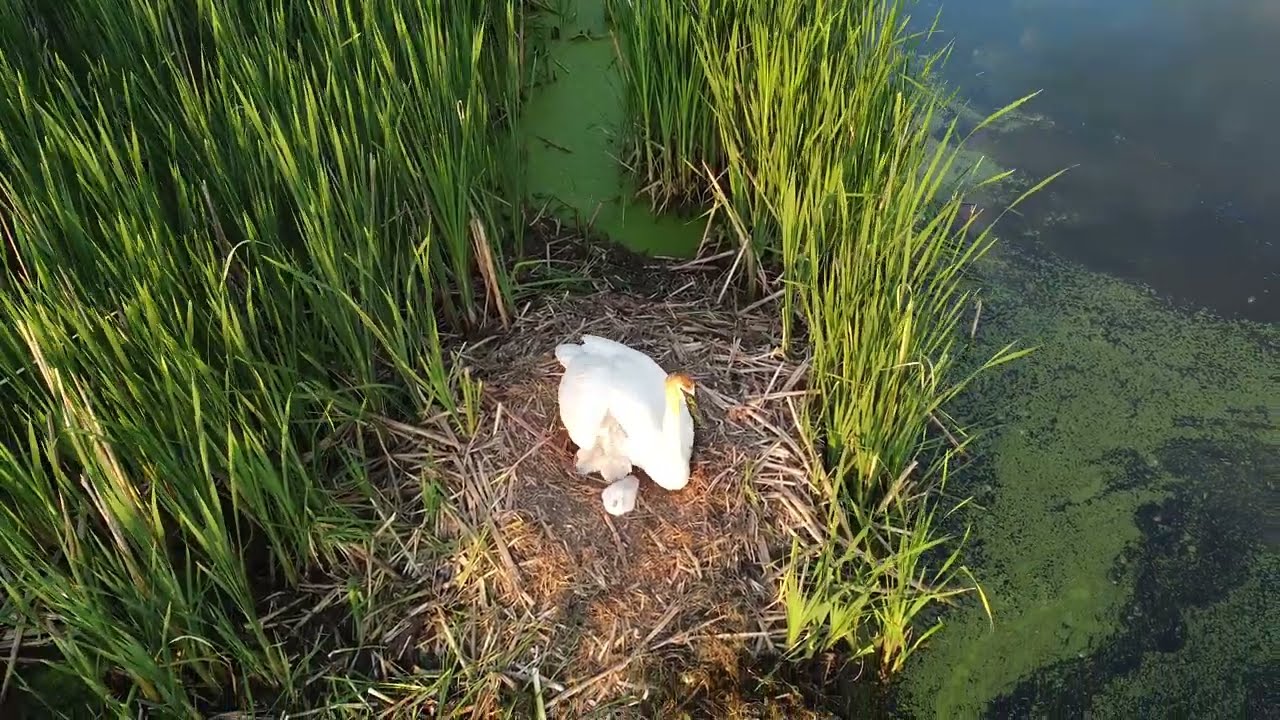This photograph captures a serene marshy area featuring a white bird, possibly a swan, nestled in a well-constructed nest. The bird, which has a distinguishing black bill and an orange-yellow head, appears to be guarding several chicks that are harder to discern due to their brownish-gray coloration blending into the surroundings. The nest itself is composed of brown shrubs, dirt, and sticks, and is situated within tall green grasses that provide a natural enclosure. To the right of the nest, the swampy water is murky and covered with green algae, adding to the idyllic yet wild setting. The image showcases the bird amid its natural habitat, underscored by the lush greenery and the moss-laden, dark water nearby.